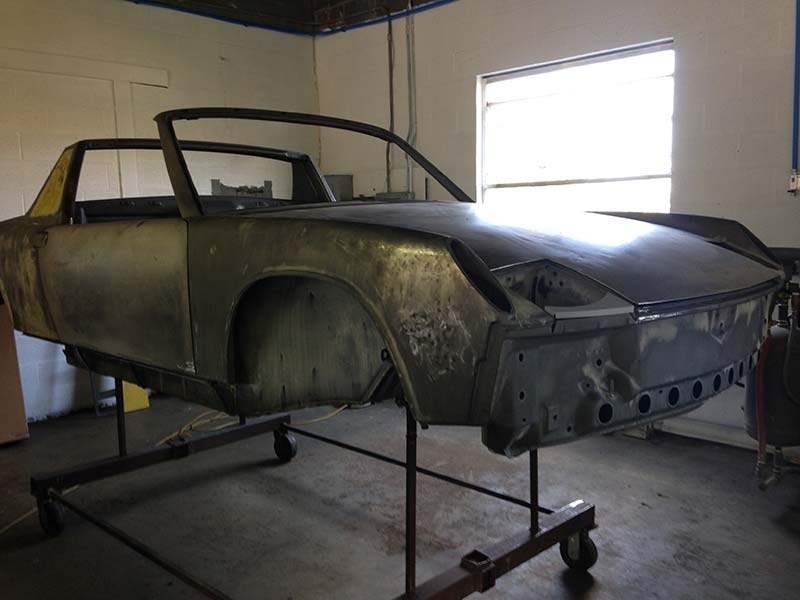This image captures the interior of a garage workshop. At the center of the photo is the stripped-down frame of a vintage sports car, devoid of wheels and an engine, resting on a mobile metal rack. The frame's metallic surface shows signs of wear, indicative of its age. Below the car, the concrete floor appears worn and slightly messy, with a yellow cord lying towards the back. In the upper right corner of the image, a window allows natural light to pour into the space, illuminating the scene. The background features a white concrete wall with vertical piping on the left side, adding an industrial touch. The overall ambiance suggests a dedicated workspace for vehicle restoration or maintenance.